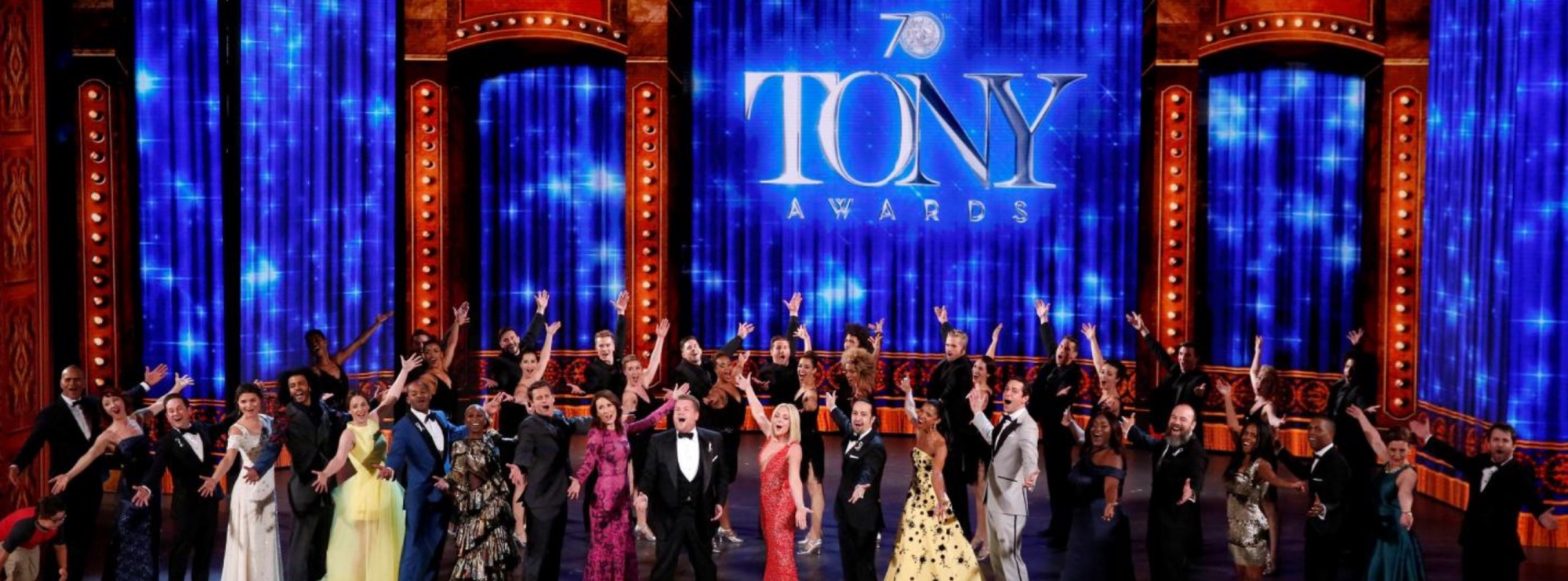This vibrant color photograph captures a dynamic moment from the 70th Tony Awards, showcasing a grand stage filled with multiple people dressed in elegant evening wear. Center stage, James Corden stands prominently in a classic tuxedo, surrounded by a multitude of celebrities and actors, all impeccably dressed in fancy suits and dresses. The performers are in the midst of a grand finale, their arms outstretched and one arm raised high in unison, suggesting the climactic end of their number. 

The backdrop of the stage is visually striking, featuring a large video screen wall adorned with draping blue lines that sparkle with white glistening stars. Flanking the background are two large, slightly rounded archways, each embedded with vertical lights that ascend up the sides and cross the tops, adding to the stage's majestic illumination. The sleek, glossy black stage floor reflects the performers and the dazzling lights above. Dominating the center of this opulent backdrop is a sign that reads "70 Tony Awards" in shiny, glossy silver text, commemorating the event’s milestone year. The overall effect is one of grandeur and celebration, capturing the essence of one of Broadway's most prestigious nights.